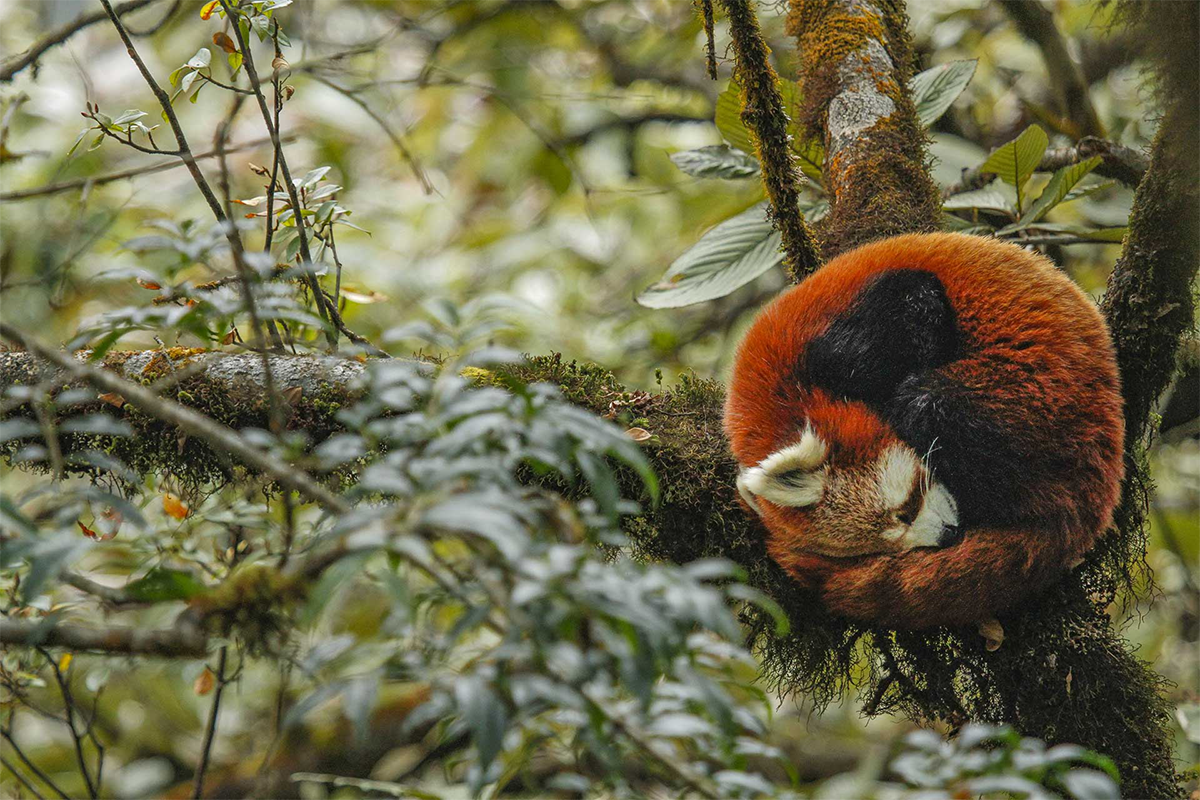A majestic, towering tree with a sturdy, brown trunk and sprawling branches adorned in thick moss stands prominently against a light gray sky. The tree's ample green leaves create a lush canopy, providing a verdant backdrop. Among the branches on the right side, a small red fox is curled up peacefully, asleep. The fox has a distinctive white face with a brown stripe running across its eyes. Its ears are mismatched—one is a blend of white and light brown, while the other is a rich reddish color. The fox's predominantly red fur is accented with black patches along its midsection and black-tipped feet, adding contrast to its vivid coat.